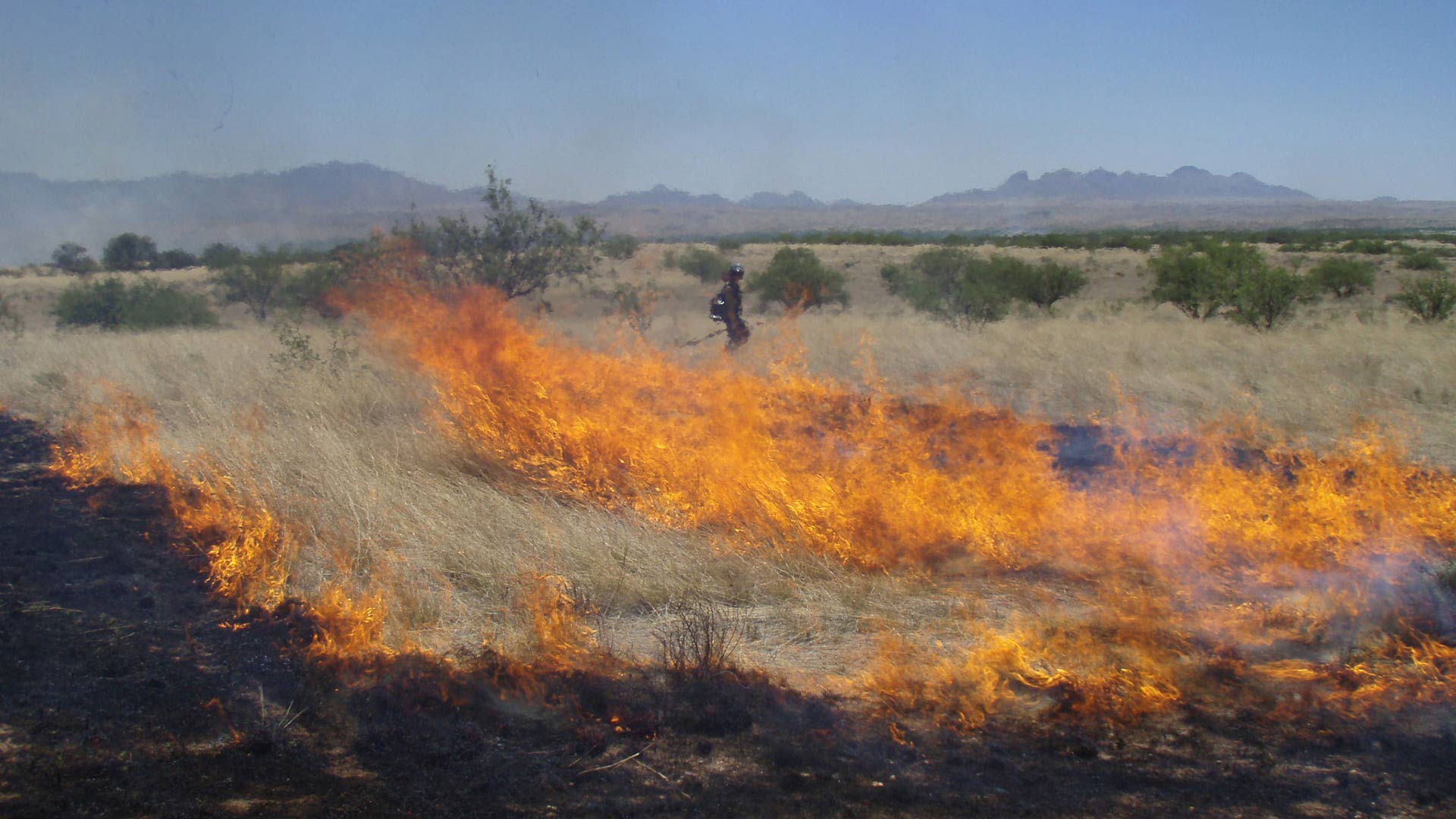The image captures an outdoor scene of a brush fire engulfing a dry, grassy field. The foreground is dominated by light brown, thin grasses, many of which are already burning, creating a line of golden-red flames stretching from the right to the left side of the image. A noticeable, larger swath of more intense flames is spreading from the right towards the left of center, with blackened, charred ground beneath them. Scattered around the field, particularly in the background, are smaller green shrubs and bushes, contrasting against the dry landscape. In the far distance, sandy ground transitions to a horizon of mountainous or hilly regions under a bright blue sky, with what looks like a heat haze overlaying it. Amidst the flames, a figure can be seen in the center of the image, dressed in dark protective gear and wearing a helmet, possibly holding a flamethrower or a similar tool, adding a compelling human element to the scene. This figure, presumably a firefighter, is positioned beyond the flames, seemingly battling or controlling the blaze. The entire scene gives a sense of urgency and the relentless advance of the fire across the barren, drought-stricken terrain.